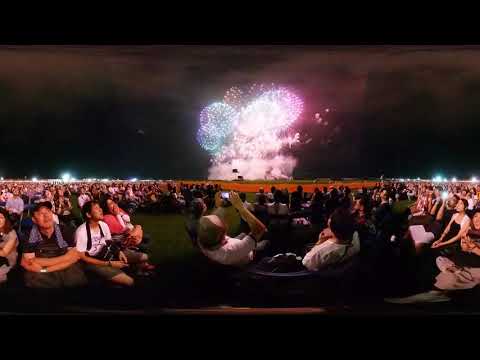A large crowd has gathered in a park on a hot summer night to watch an impressive fireworks display. The sky is pitch black, providing a stark backdrop for the vibrant bursts of color, including blues, pinks, greens, and purples. The fireworks, which appear to be in circular shapes, are accompanied by clouds of smoke and are drawing awe and excitement from the audience. Most people are seated, some with short sleeves and shorts, indicative of the warm weather. Many spectators are capturing the moment with their phones, their screens and camera flashes visible in the distance. The festive atmosphere suggests a celebration, possibly the 4th of July, with hundreds to possibly a couple thousand people present, all mesmerized by the ongoing, spectacular light show.